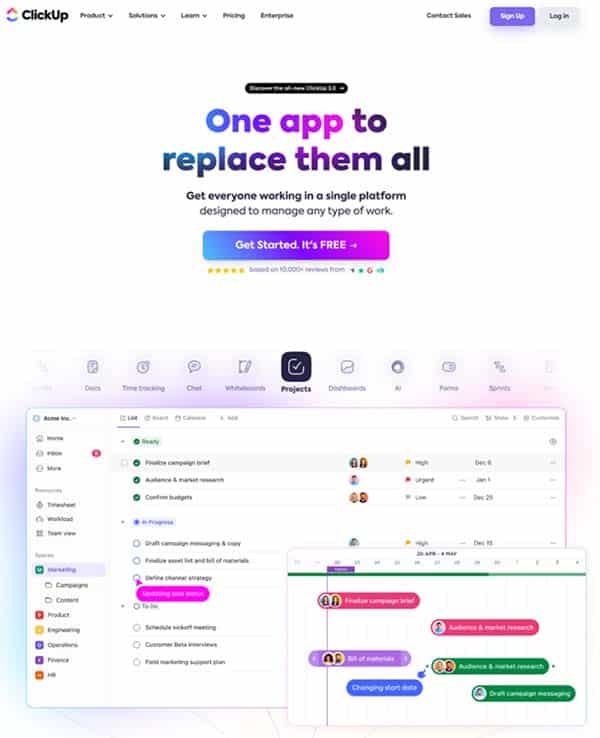This illustrated image depicts the homepage of ClickUp's website. Dominantly displayed in bold text is the slogan, "One app to replace them all," emphasizing the platform's capability to consolidate various work management tools into one application. Below this tagline, promotional text invites users to "Get everyone working in a single platform designed to manage any type of work."

A prominent button, shaded with a gradient of purple and pink hues and labeled "Get Started, It's Free," encourages visitors to begin using the platform without any initial cost. This call-to-action is visually striking, drawing immediate attention.

The platform's broad range of functionalities is highlighted through tabs labeled: Docs, Time Tracking, Chat, Whiteboards, Projects, Dashboards, AI, and Forms, showcasing the diversity of tools integrated into ClickUp. Above these tabs, a note indicates that the platform is highly rated, with a user base that has provided "Based on 10,000 reviews."

To personalize the experience, the image features small circular profile pictures of various users, including two women and one man, reflecting a diverse and engaged community. Specific buttons cater to different organizational departments and functions, listing options such as Campaigns, Content, Product, Engineering, Operations, Finance, HR, and Campaign Brief, thereby showcasing the platform's versatility across different business needs.

At the very top of the image, a distinct purple button marked "Sign Up" offers another prompt for users to join the platform, ensuring the call-to-action remains accessible from multiple points on the webpage.